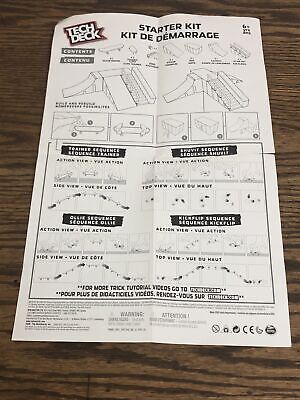This image illustrates a detailed instruction manual for assembling a Tech Deck Starter Kit. The black-and-white page, printed in both English and French, features the title "Starter Kit" and "Kit de Démarrage" prominently at the top. In the upper left corner, "Tech Deck" is written in distinctive white font against a black background. The manual outlines approximately eleven distinct steps to assemble various components, including ramps and staircases, vital for setting up the deck. The instructions are broken down into several segments, some enclosed within four black boxes with white text, providing detailed explanations on installation and usage. Additionally, the page is scattered with various symbols to aid understanding. The manual is resting on a wooden table, adding a natural texture to the background. There's fine print located at the bottom of the page as well.